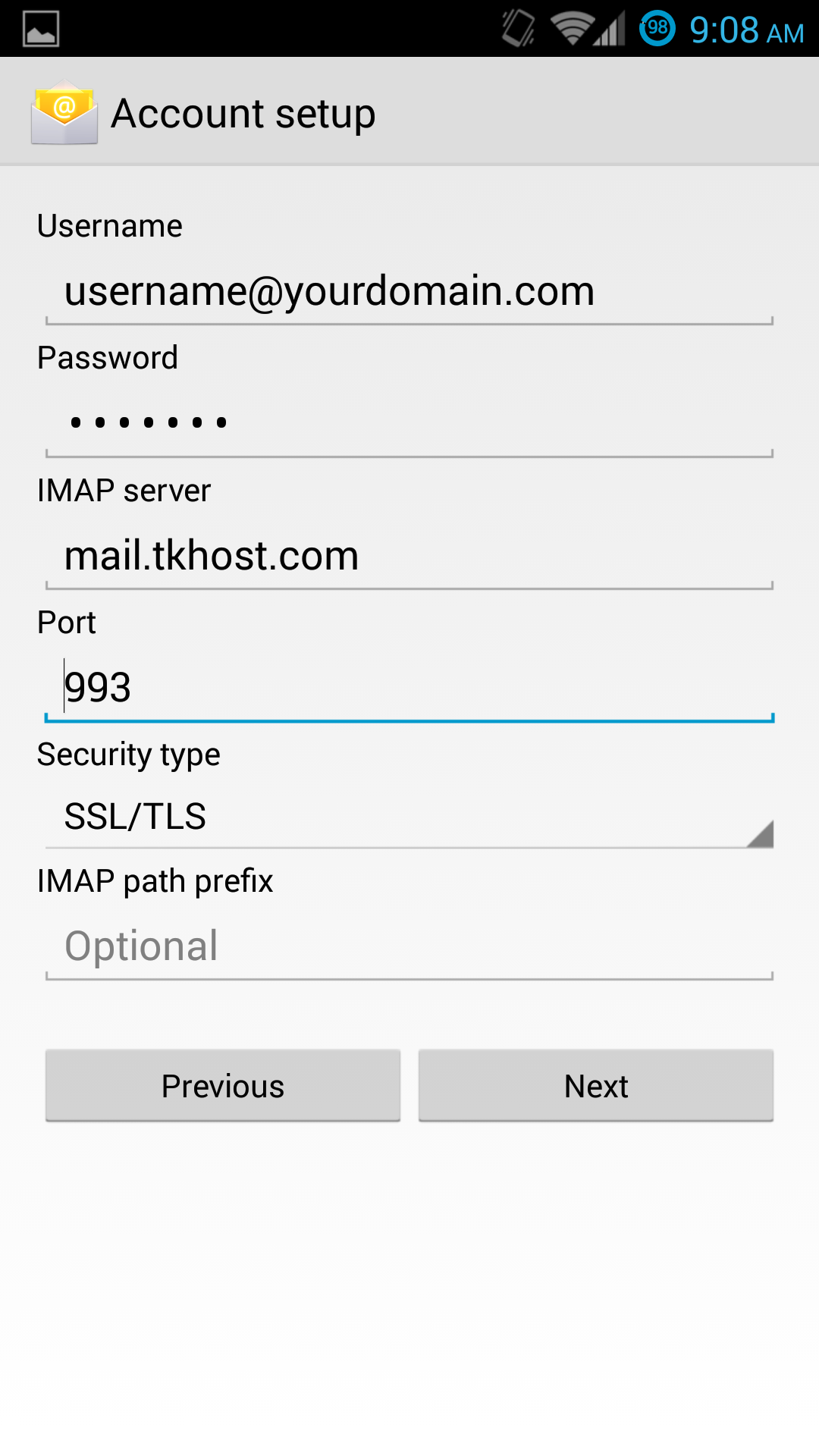This image depicts a screenshot of a phone interface displaying an account setup menu. At the top of the screen, it prominently reads "Account Setup," indicating the current process being undertaken. On the top right corner, the time is shown as 9:00 AM with baby blue lettering, making it stand out against the black bar. The Wi-Fi and connection symbols are also visible, signifying an active internet connection.

The main section of the screen features various fields that need to be filled out to complete the account setup. The first field is labeled "Username" with an example entry, "username@yourdomain.com". Beneath this, the password field is represented by dots for security. Following this is the "IMAP server" section, which lists "mail.tkhost.com". The subsequent fields include the port number, "Port 993," the security type, "SSL/TLS," and the "IMAP path prefix," which is noted as optional and left blank in this instance.

The bottom of the screen features two buttons: “Previous” on the left and “Next” on the right, both in gray with black lettering. The overall color scheme of the interface is predominantly gray with accents of black and blue, giving it a clean and organized appearance. This setup seems designed to help users configure their email accounts on their phones, ensuring they can access their emails seamlessly.